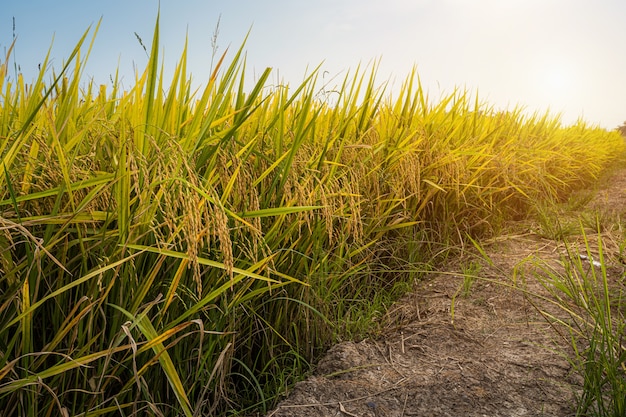This is a detailed color photo taken outdoors during the daytime. The image captures an overgrown dirt path running through what seems to be a field. The narrow, cracked brown dirt path is flanked by tall, green, and yellow stalks—possibly crops like wheat—reaching nearly the height of the person who took the picture. On the left of the path, lush green grass grows, while the right side features a blend of tall and short grasses, with some dried and dead patches scattered throughout. The path appears to have a rut down the middle, likely from a tractor. The sky above is a muted blue, fading into white, particularly intense in the far right corner, suggesting a high sun. The colors in the photograph prominently feature various shades of green, yellow, and white, creating a serene yet slightly desolate atmosphere.